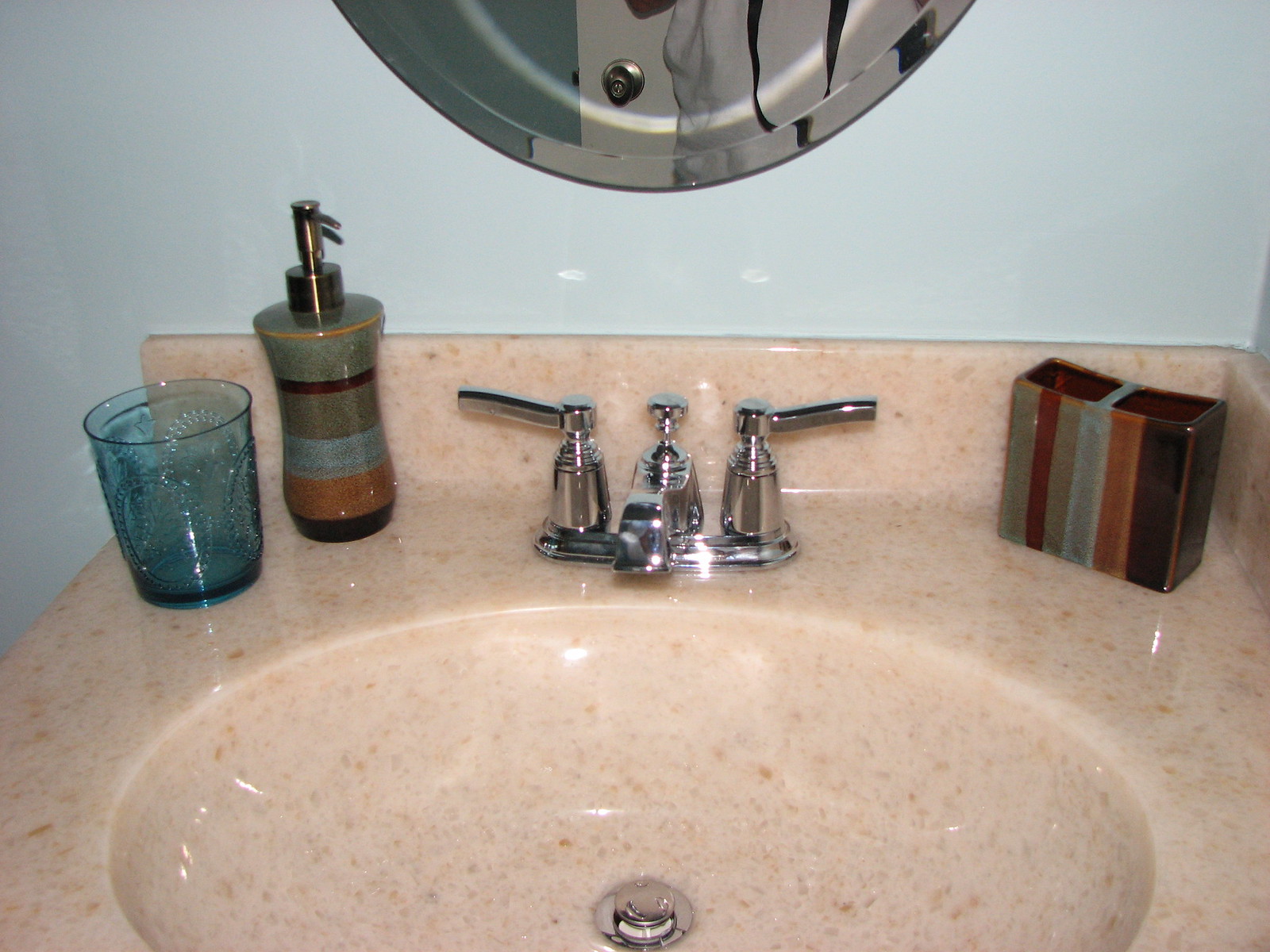The image showcases a well-appointed bathroom sink integrated into a matching beige countertop with subtle specks of gray and darker tan accents. On the counter sits an elegant set of hand soap and soft soap pumps, adorned in a color scheme of dark beige, maroon, and dark blue, which is mirrored in the vertical lines decorating the adjacent toothbrush holder. The sink's spigot and contemporary hot and cold handles appear to be brand new, adding a modern touch. Above the sink, a mirror framed in the same hues as the soap dispenser and toothbrush holder enhances the cohesive design. To the left of the soap dispenser, a blue drinking glass with a decorative design adds a pop of color. The bathroom wall is painted a soothing, very light blue with a green undertone, harmonizing beautifully with the entire decor.